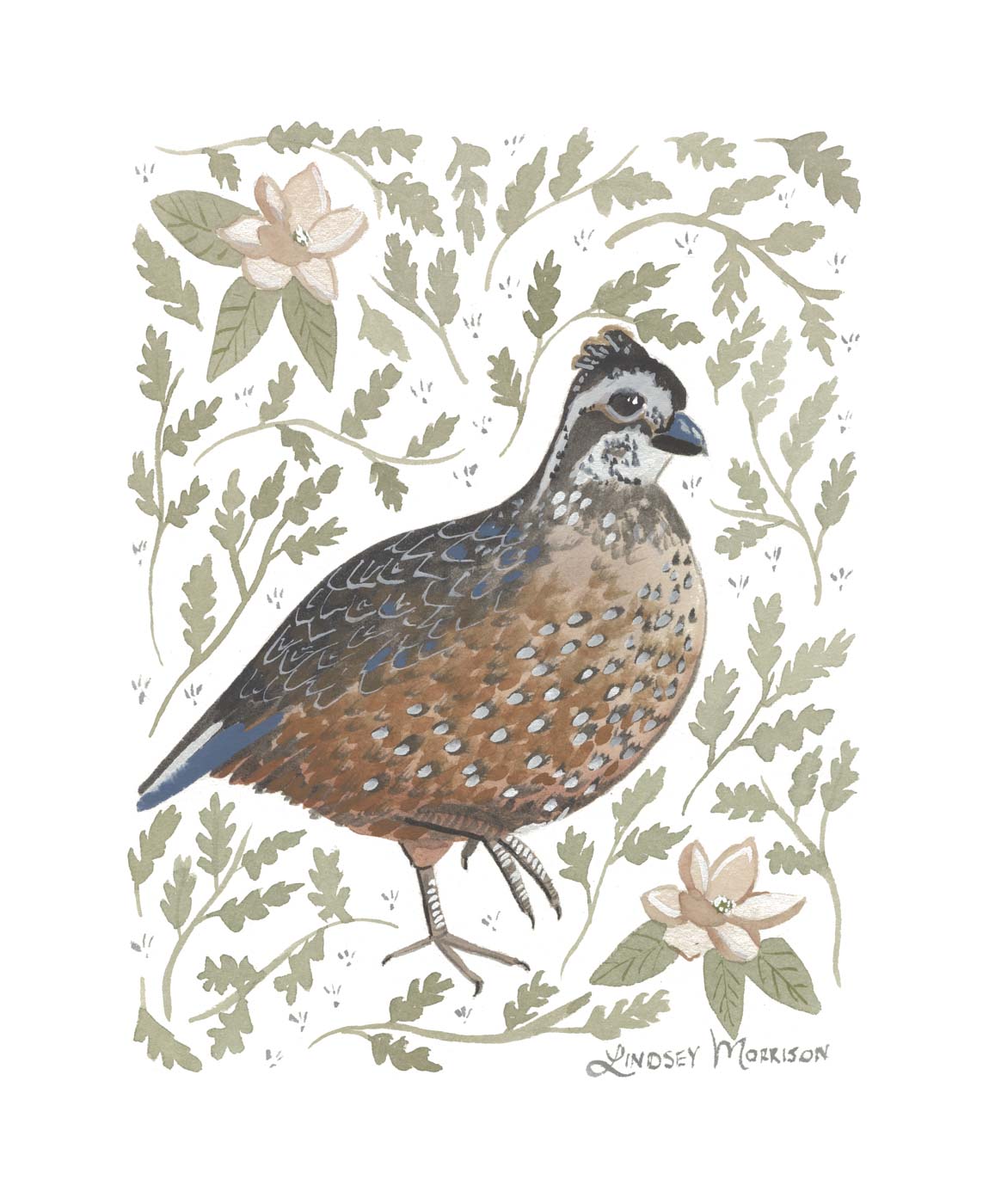This is a detailed painting in muted watercolors by Lindsay Morrison, prominently featuring a pheasant at its center. The bird is depicted with a nuanced brown breast adorned with gray spots, transitioning to darker brown feathers on its back and a mix of brown, gray, and blue in its tail feathers. The pheasant, which has a distinctive white throat and three short feathers atop its dark crown, is shown with one claw lifted in a delicate pose. Its head displays a blend of lighter and darker grays, some brown patches, and a black beak.

Surrounding the pheasant are numerous slender branches with tiny leaves, rendered in a soft, muted green, creating a delicate frame for the bird. In the top left and bottom right corners, the artist has added larger, pointed leaves alongside pale pink flowers, adding a splash of subdued color. The artwork is signed "Lindsay Morrison" in the lower right corner in a subtle charcoal hue. The background is a clean white, allowing the details of the bird and foliage to stand out vividly.